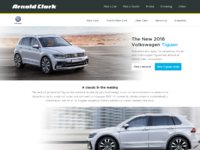This image appears to be a screenshot of a car-related website. The image is somewhat blurry and appears to be taken from a distance, making some details hard to discern. 

In the bottom left corner, there is a white blurred area that cuts off part of the screen. Adjacent to this white blur is an image of a modern, four-door white hatchback car. The car is oriented to the left if you are facing the screen.

In the background, there is a building with discernible black spots, likely windows or ledges. At the top of the image, there's a black banner which might contain text—possibly names, though the exact details are unclear but it might be related to "Arnold Kirk" or a similar name.

On the right-hand side of the image, there are about five selectable options, possibly navigation or menu items. Toward the bottom right, another image of the same car is visible, this time showing the front face of the car angled to the right.

Additionally, there is a title at the top of an article, presumably mentioning "Volkswagen". Below the title, there is a paragraph of text and two buttons. One button is highlighted white, and the other in an aqua blue color.